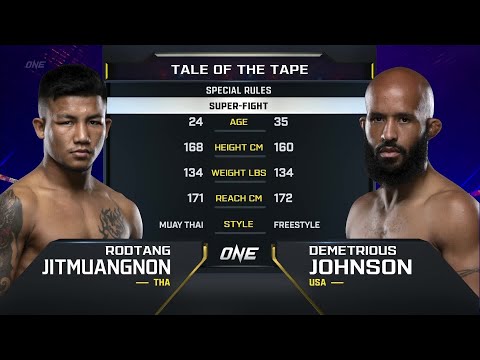This promotional image, set up as a title card for a boxing or fighting match, is dominated by detailed statistics of two fighters. The top of the chart features the headings "Tale of the Tape" in white text, "Special Rules," and "Super Fight" in black text. On the left side stands Rodthang Jitmuangnon from Thailand, aged 24, with a height of 168 centimeters, a weight of 134 pounds, a reach of 171 centimeters, and expertise in Muay Thai. He is depicted as shirtless with short black hair and a tattoo on his right arm and chest. On the right side is Demetrius Johnson from the USA, aged 35, standing 160 centimeters tall, weighing 134 pounds, with a reach of 172 centimeters, and practicing freestyle fighting. He is shown as a shirtless black male, sporting a black beard and mustache, and completely bald. The image at the center highlights the fighters' stats side by side, conveying a sense of anticipation for the upcoming bout.